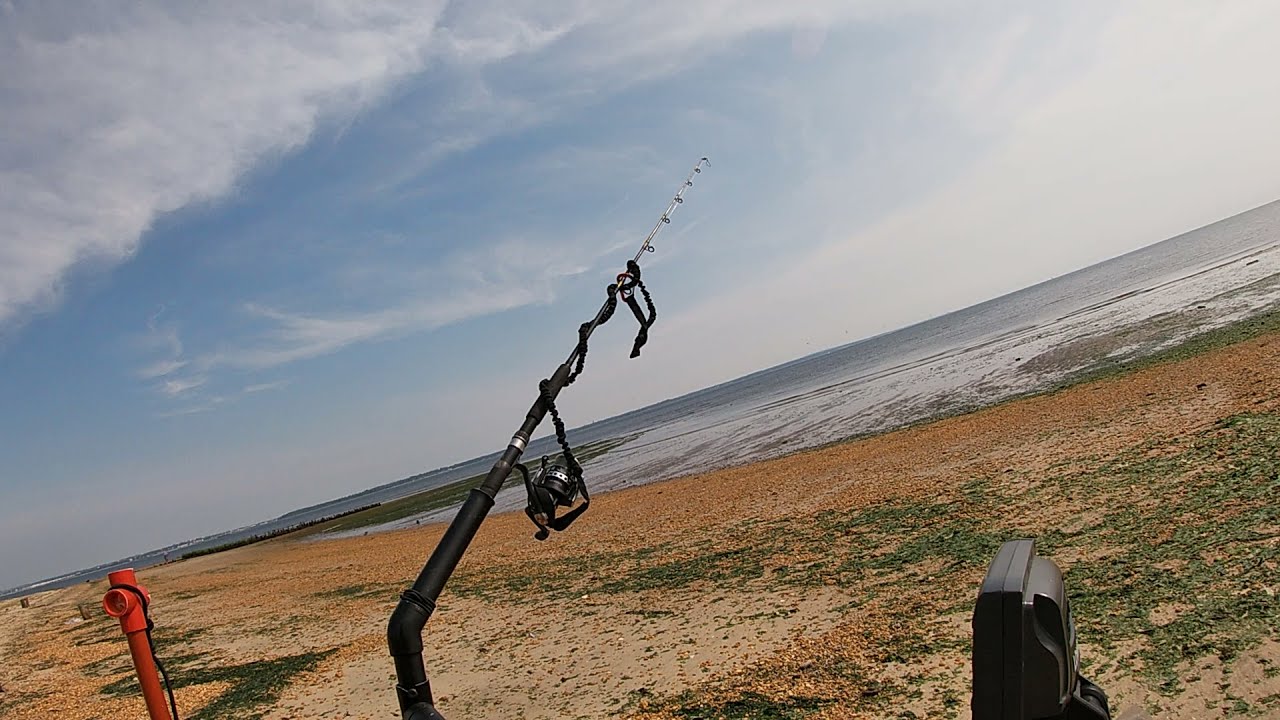The photograph captures a serene beach scene viewed from approximately 40 to 50 feet away from the shoreline. Dominating the foreground, a black and silver fishing rod is prominently propped up using a black metal holder, with the rod angled towards the ocean. The fishing rod is unattended and no fishing line is visible. To the image's right and near the base, there is what appears to be seaweed or another indistinct black object on the sandy shore. Also noticeable is a red pipe with a black wire coiled on it, positioned to the left of the scene, part of which is obscured within the sand. The beach itself displays a mix of brown sand and small rocks, dotted with patches of green seaweed. The distant water changes from a dark blue to grayish hue under the expansive sky, which is painted with scattered white clouds. The horizon in the background appears slightly slanted, adding a dynamic element to the tranquil seascape.